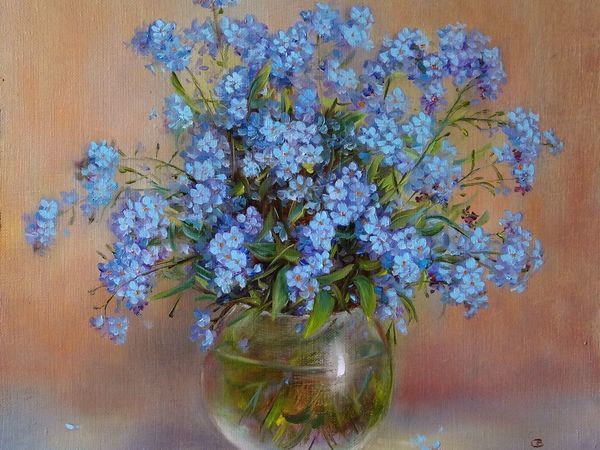The image features a highly realistic oil painting of a bouquet of blue, five-petaled flowers, each blooming with a variety of stems and leaves. They are artistically arranged within a clear, fishbowl-like vase whose circular body is topped off slightly below the rim. The transparency of the vase allows an intimate view of the stems and leaves submerged in water, with the water line skillfully depicted by the artist. This detailed scene is set against a moody, rusty orangey-red background resembling a vintage wall, enriching the depth and warmth of the overall composition.